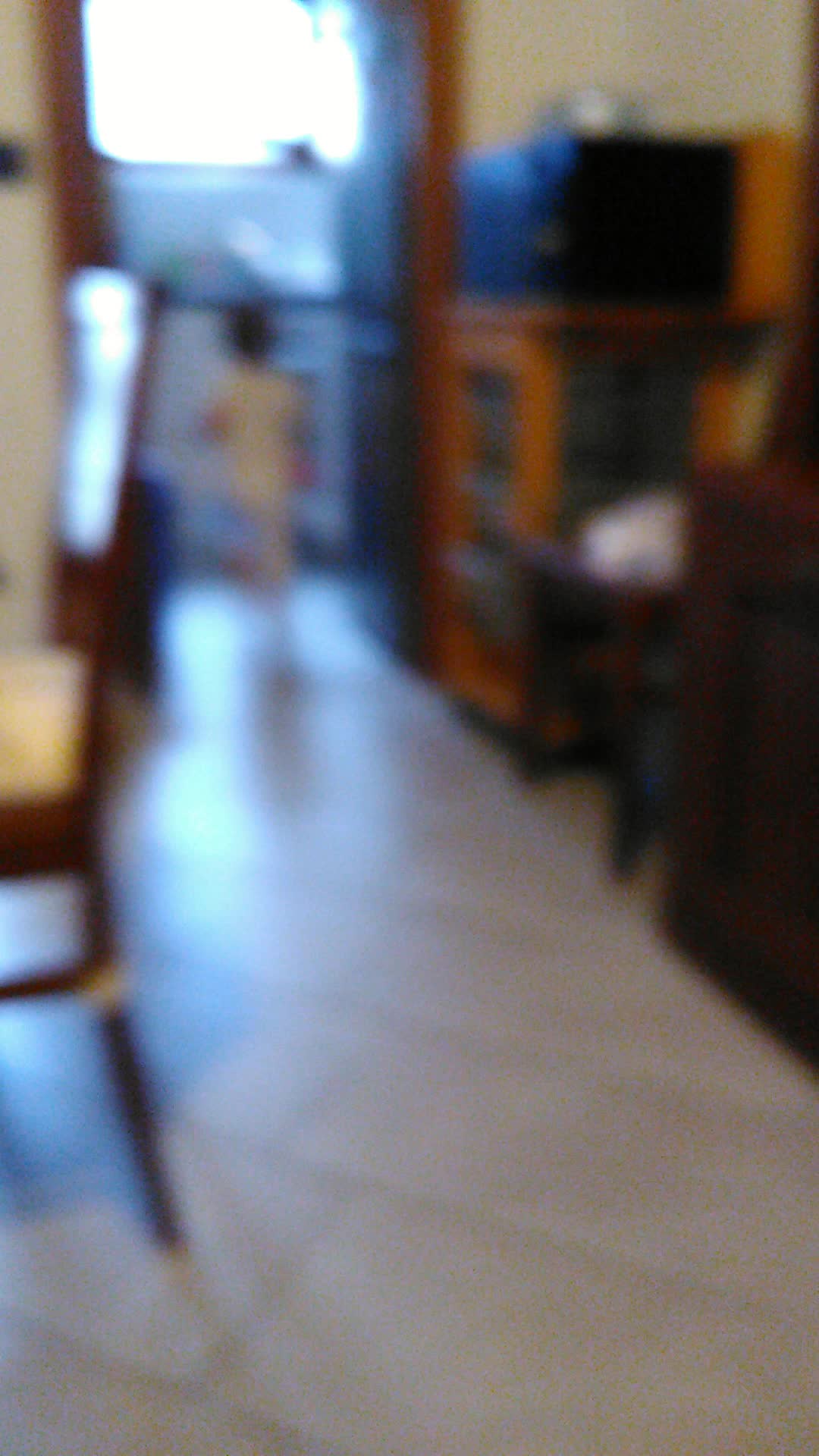This color, portrait-format photograph depicts the blurry interior of a family home, characterized by white tile floors and white walls. The shot appears to be taken from the junction between a living room and a dining room, indicated by the presence of a wooden doorway in the background. In the foreground, a brown wooden chair with a white cushion is partially visible on the left. Along the right-hand side, a light brown cabinet with a black object, possibly a piece of technology, on top can be seen, accompanied by another dark brown piece of furniture and a chair. A small child, dressed in off-white clothing and with dark hair, is seen walking away from the viewer through the doorway, enhancing the sense of depth in the photograph.